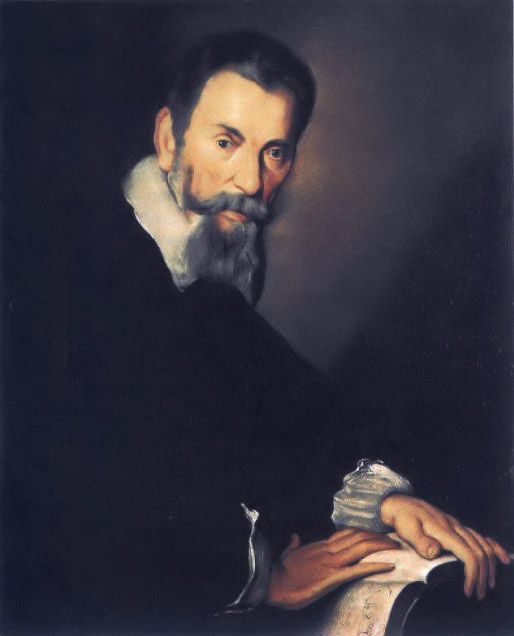This painting depicts an elderly man, likely in his 70s, with dark, graying hair, a gray mustache, and a long gray beard or goatee. His olive-toned skin accentuates his deep brown eyes, which gaze contemplatively into the distance. The man is dressed in a white collared shirt beneath what appears to be a black sweater or cloak, featuring white cuffs at the sleeves. He rests his hands gently on an open book with visible white pages. The background is predominantly dark, but a lighter area in the center illuminates his face and attire, suggesting a focused light source. The overall effect is one of solemnity and introspection, with the man appearing to pose thoughtfully for the artist.